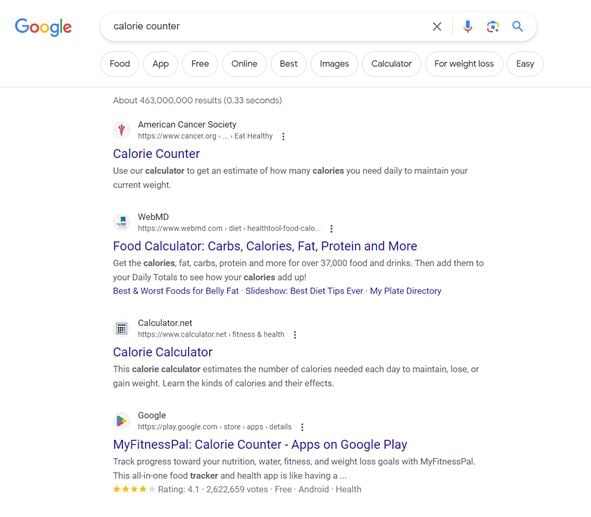The image depicts a Google search results page. In the upper left corner, the word "Google" is displayed in its signature multi-color font. Below it, a gray rectangular search bar expands slightly at the ends, resembling circles. Inside the search bar, text appears on the left, while the right side contains an "X" icon, a microphone icon, an indistinguishable colorful symbol, and a magnifying glass icon.

Below the search bar, there is a list of nine differently labeled, rounded rectangular tabs displayed horizontally. A light gray line appears beneath these tabs, followed by a block of smaller text written in gray.

Further down, a small, partly visible symbol in red and purple is present, followed by a line of black text. A section title in blue indicates "Calorie Counter," with additional descriptive text underneath. Adjacent to a white and blue icon, the phrase "Food Calculator: Carbs, Calories, Fat, Protein, and More" is highlighted in blue or purple, accompanied by explanatory text in black.

Lastly, the page features a triangular multicolored symbol with accompanying text. Under this, the phrase "MyFitnessPal: Calorie Counter – Apps on Google Play" is prominently displayed in blue or purple. The description includes additional black text and yellow stars, followed by more black text.